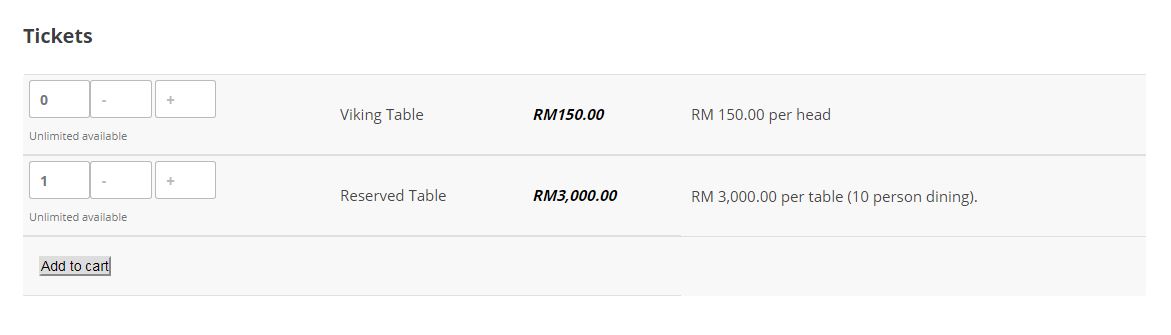This image depicts a section of a ticket-purchasing page. In the upper left corner, "Tickets" is prominently displayed in bold black font. The background features a light gray color, and various sections are delineated by horizontal lines.

The first section includes three horizontally aligned white boxes: the first box displays "0," the middle box shows a dash ("-"), and the last box contains a plus sign ("+"). Centered within this section is the text "Viking Table," followed by a tabulated bold font indicating "RM150.00." Another tab specifies "RM150.00 per head."

Below this, another set of white background boxes features the first box with "1," followed by a hyphen ("-"), and the last box with a plus sign ("+"). A tab follows, leading to the text "Reserved Table." Subsequent tabs reveal "RM3000.00" in bold font and "RM3000.00 per table," with a note in parentheses, "(per person dining)."

The section ends with another horizontal line, beneath which the background turns a darker gray color, and the text "Add to Cart" appears underlined.